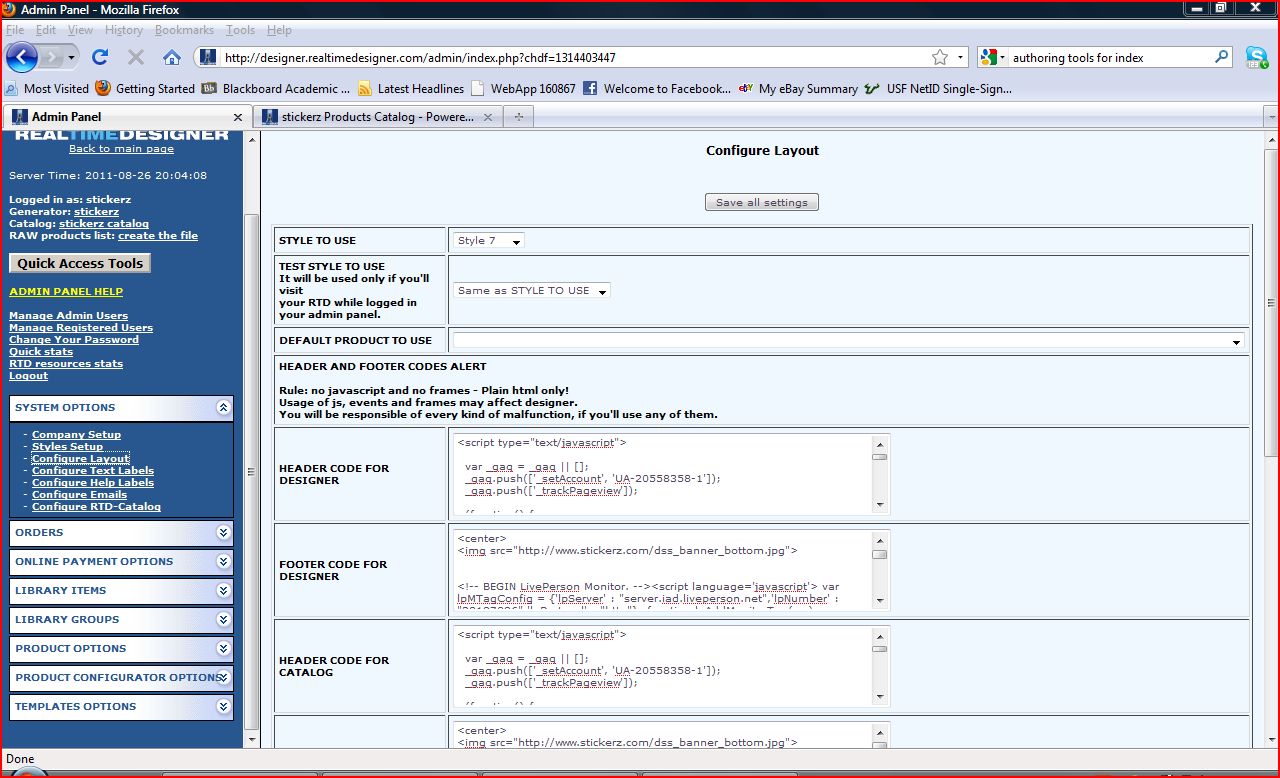The image displays the admin panel of the Realtime Designer website, accessed via Mozilla Firefox. The URL in the browser's address bar is "designer.realtimedesigner.com/admin/index.php". The page is titled "Realtime Designer" and includes options such as "Back to Main Page," "Server Time" (2011-08-26 20:04:08), and "Logged in as: StickerZ". 

The left sidebar features an extensive menu with sections including "Generator," "StickerZ Catalog," "Raw Product List," "Create File," and "Quick Access Tools." Additionally, there are links for "Admin Panel Help," "Manage Admin Users," "Manage Registered Users," "Change Your Password," "Quick Stats," "RTD Resource Stats," and "Log Out." 

Further configuration options in the sidebar include "System Options," "Company Setup," "Style Setup," "Configure Layout," "Configure Text Label," "Configure Help Label," "Configure Emails," and "Configure RTD Catalog." 

Below the configuration options, administrative sections for handling "Orders," "Online Payments," "Options," "Library Items," "Library Groups," "Product Options," "Product Configure Options," and "Template Options" are present. 

In the main content area of the page, there is a central heading labeled "Configure Layout," along with a button to "Save All Settings."